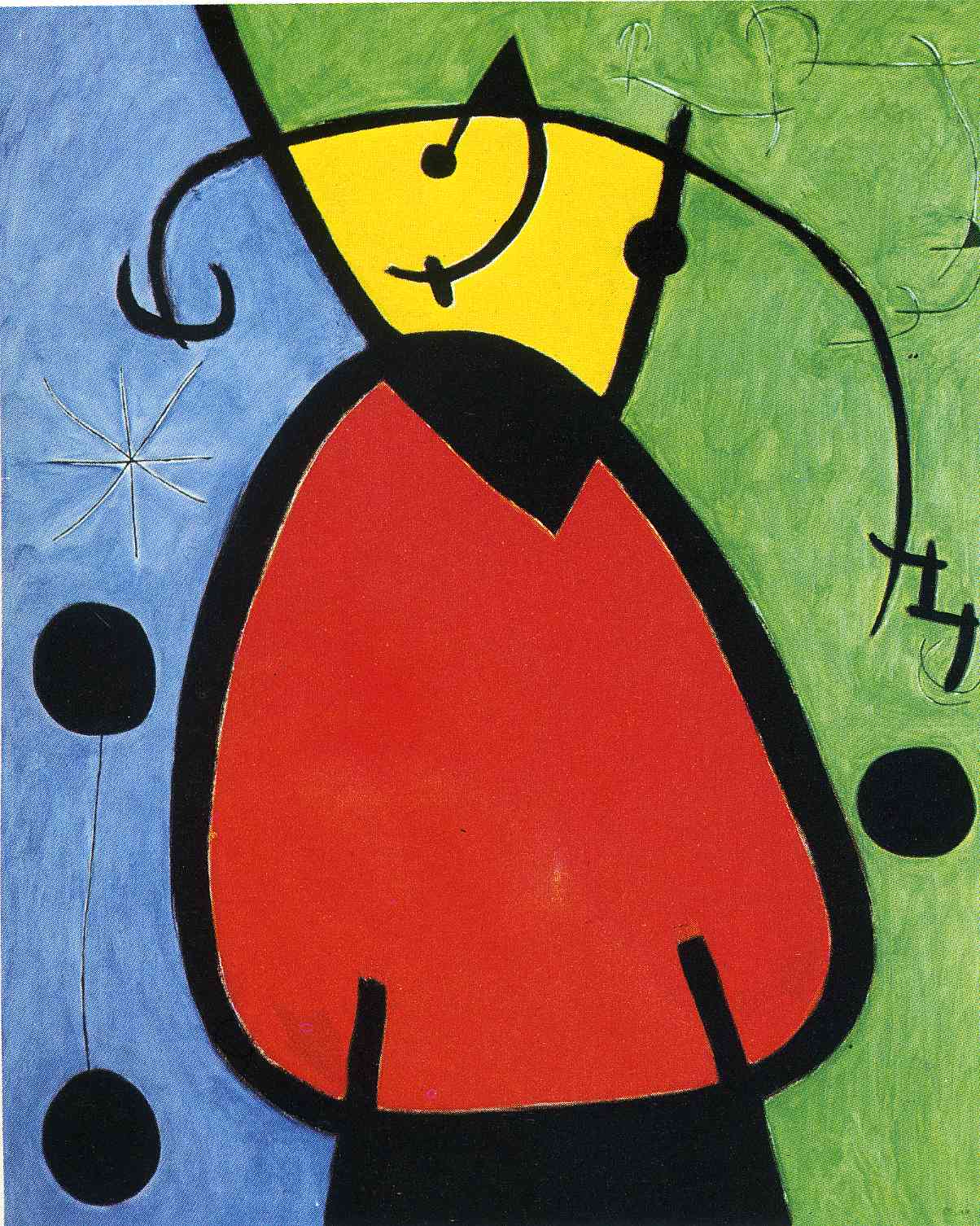This artwork is a vibrant and modern painting known as "The Birth of Day" by Joan Miro, characterized by its simplistic yet unique design on textured canvas. Dominated by primary colors, the right side of the piece is awash in green, while the left is a striking blue. At the center, a red, oval-like form with black dots emerges, its bottom extending into what appear to be legs or arms. Overlaying this central figure is a black triangle with rounded edges, from which a black square extends downward. Atop the triangle lies a yellow rectangular shape adorned with facial features, including a smile and an eye, giving it a whimsical, almost ladybug-like appearance. To the left, two black circles connected by a line sit beneath a star shape, while on the right, a single black circle is accompanied by an M-shaped form and a hook-like appendage protruding through the yellow shape. Additionally, slender black lines curve elegantly across the top of the painting, adding to its abstract and dynamic composition. This art piece employs rich outlines and incorporates scratches and star-like patterns, creating a multi-dimensional, engaging visual experience.